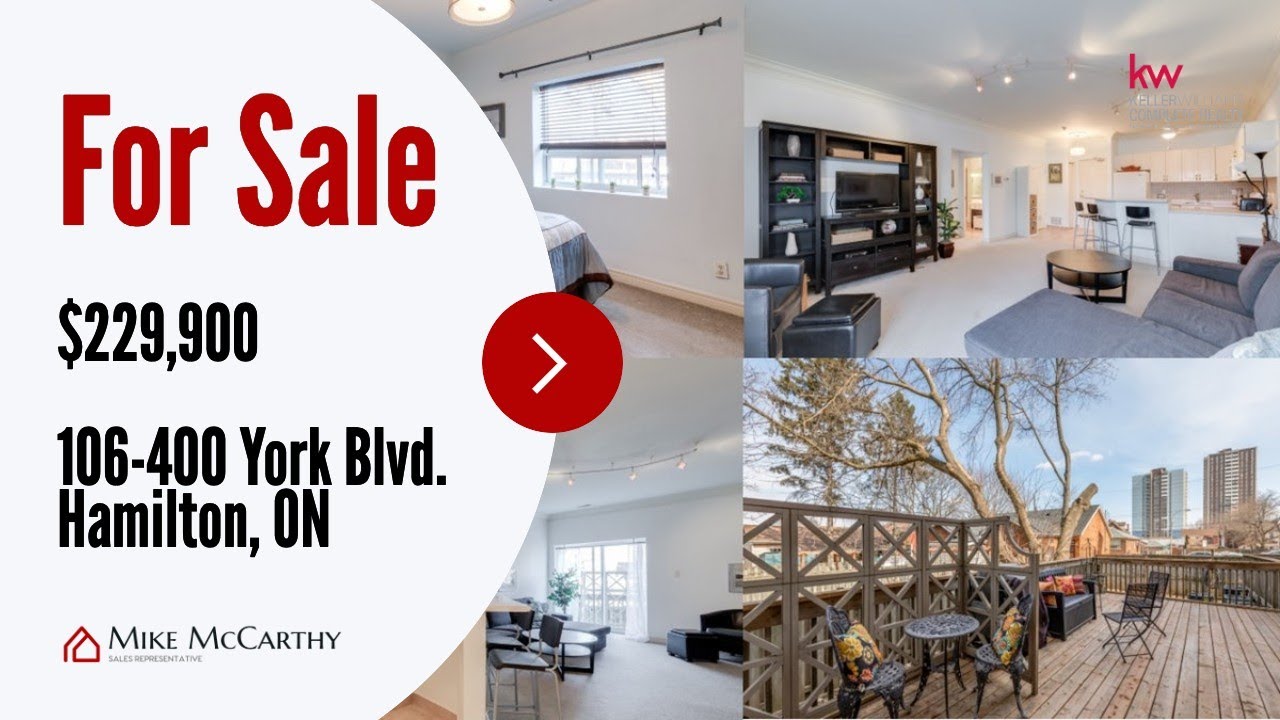For Sale: 106-400 York Boulevard, Hamilton, ON - $229,900

This advertisement showcases a home for sale, featuring both interior and exterior images prominently displayed. On the left side of the page, large red text announces "For Sale." Directly below, the price, $229,900, along with the address, 106-400 York Boulevard, Hamilton, ON, are clearly listed. 

The contact information is provided in smaller text, with "Mike McCarthy" noted beside a red house icon, followed by "Sales Representative" beneath his name. Additionally, a conspicuous red circle with a white rightward arrow appears to the right of this information.

The text and details are overlaid on two partially visible images of the home. The top image, taken inside a bedroom, reveals part of the bed, wall, and a window. The lower image displays a bit of the dining and living areas, with a large window in the background.

On the right side of the page, the layout features more unobscured photographs. The top-right image captures the home's interior, showcasing the dining area, kitchen in the background, a couch on the right, and various seating options. Beneath this, in the lower-right corner, there's a photo of a deck, complete with outdoor furniture and tall buildings visible in the distance.